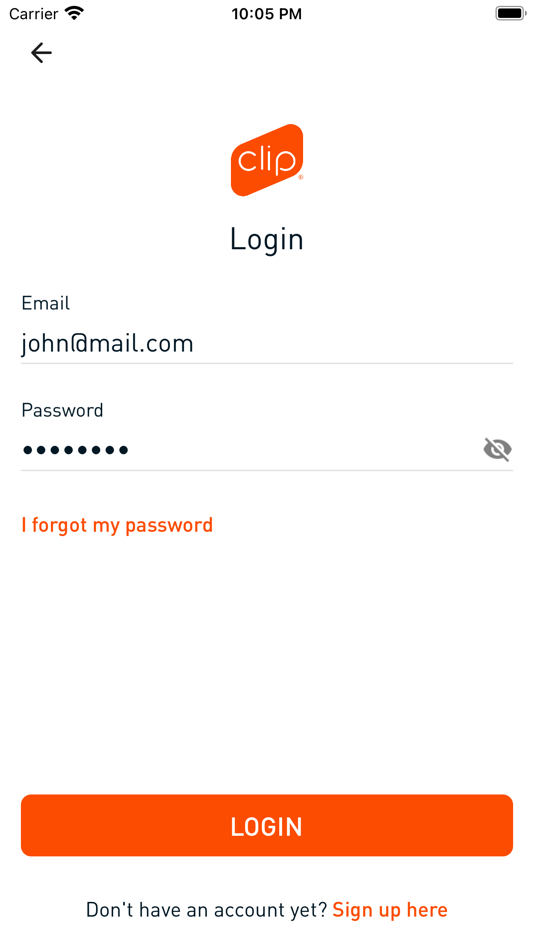The screenshot is a detailed depiction of the login screen for an app named "CLIP." The app is represented by an icon featuring an orange, slightly slanted box with white letters spelling "CLIP" centered within it. 

At the top of the screenshot, the typical phone status indicators are visible: a signal strength icon for the carrier on the left, a Wi-Fi icon next to it, the current time displayed as 10:05 PM in the center, and a battery icon on the right-hand side.

Just below this status bar, on the left, there is a back arrow pointing to the left. Next to it is the CLIP logo. Beneath the logo, the word "Login" is prominently displayed, signifying the purpose of the screen. Subsequently, there is a field labeled "Email," where the email address "john@mail.com" is typed in.

Following the email field is the "Password" field, which contains a series of eight dots, indicating the password has been entered but is obscured for security. To the right of this field is an eye icon with a line through it, signifying that the password is hidden from view.

Directly underneath the password field, there is a text link in orange that reads "I forgot my password," which users can tap if they need to reset their password.

At the bottom of the screen is an orange button with white letters that reads "Log On," which users would tap to proceed with logging in. Lastly, below this button, there is a prompt that reads, "Don't have an account yet? Sign up here," providing a link for new users to create an account.